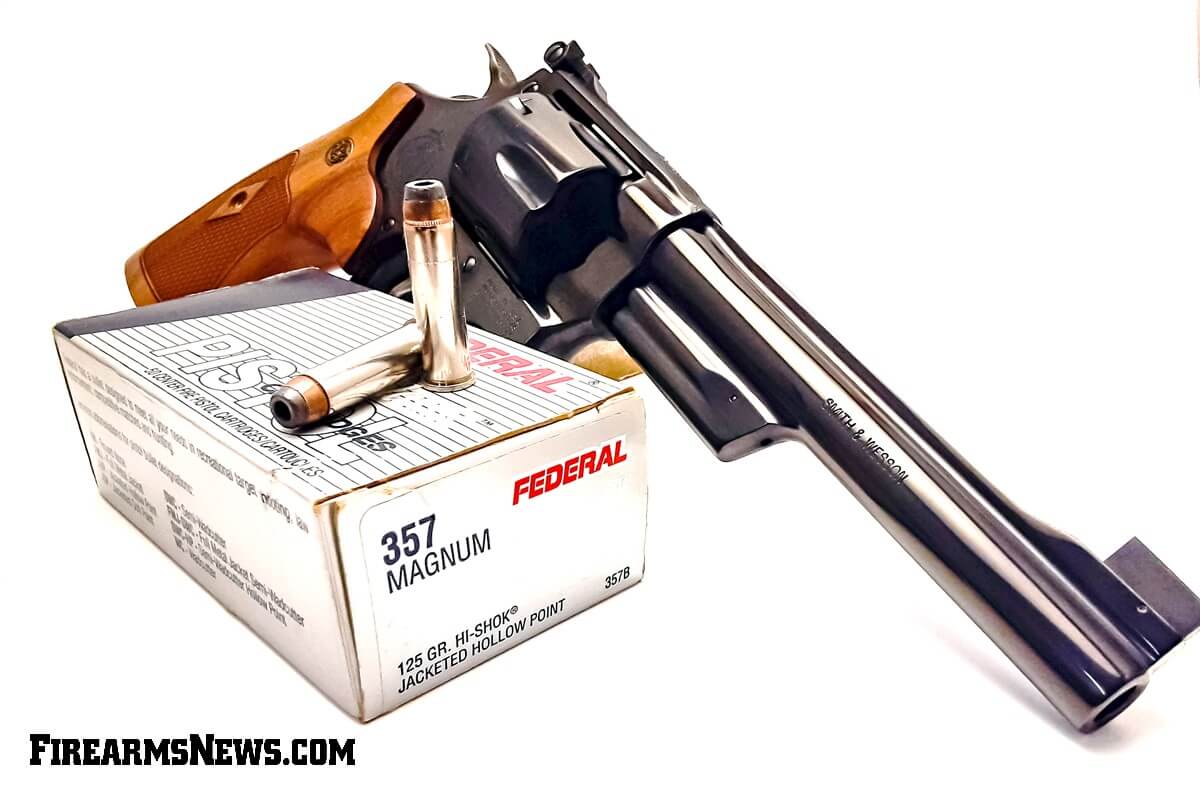The photograph captures a highly detailed and commercially styled image of a sleek revolver pistol set against a solid white background, giving the impression that it is floating in an empty white void. The image, rectangular in shape with a ratio where the top and bottom sides are twice the length of the left and right sides, is optimized for product listings typically found in online shops, websites, or catalogs.

The revolver, crafted from metal with a polished silver finish, features a wooden handle characterized by a blend of light and dark brown tones, contributing to its classic aesthetic. The gun is positioned on its handle and the front end of its barrel, which points towards the bottom right corner of the image. To keep it stable, the revolver leans against an unseen support.

Placed prominently in the foreground is a white cardboard box of ammunition, labeled with multiple lines of text. The box bears the inscription "357 Magnum" prominently on its side and "Federal" in bold red text on the top right. Additional details on the box include specifications such as "125GR High Shock Jacketed Hollow Point 357B" and a reference to "firearmsnews.com" in bold black lettering at the bottom left corner. Displayed atop this box are two silver-jacketed hollow point bullets, one standing upright and the other lying on its side.

Both the revolver and the ammunition are deliberately angled towards the bottom right corner of the image, creating a cohesive visual flow. The attention to detail, from the text on the ammunition box to the finish on the gun, highlights the quality and specifications of the products being showcased, making it an effective and detailed commercial photograph.